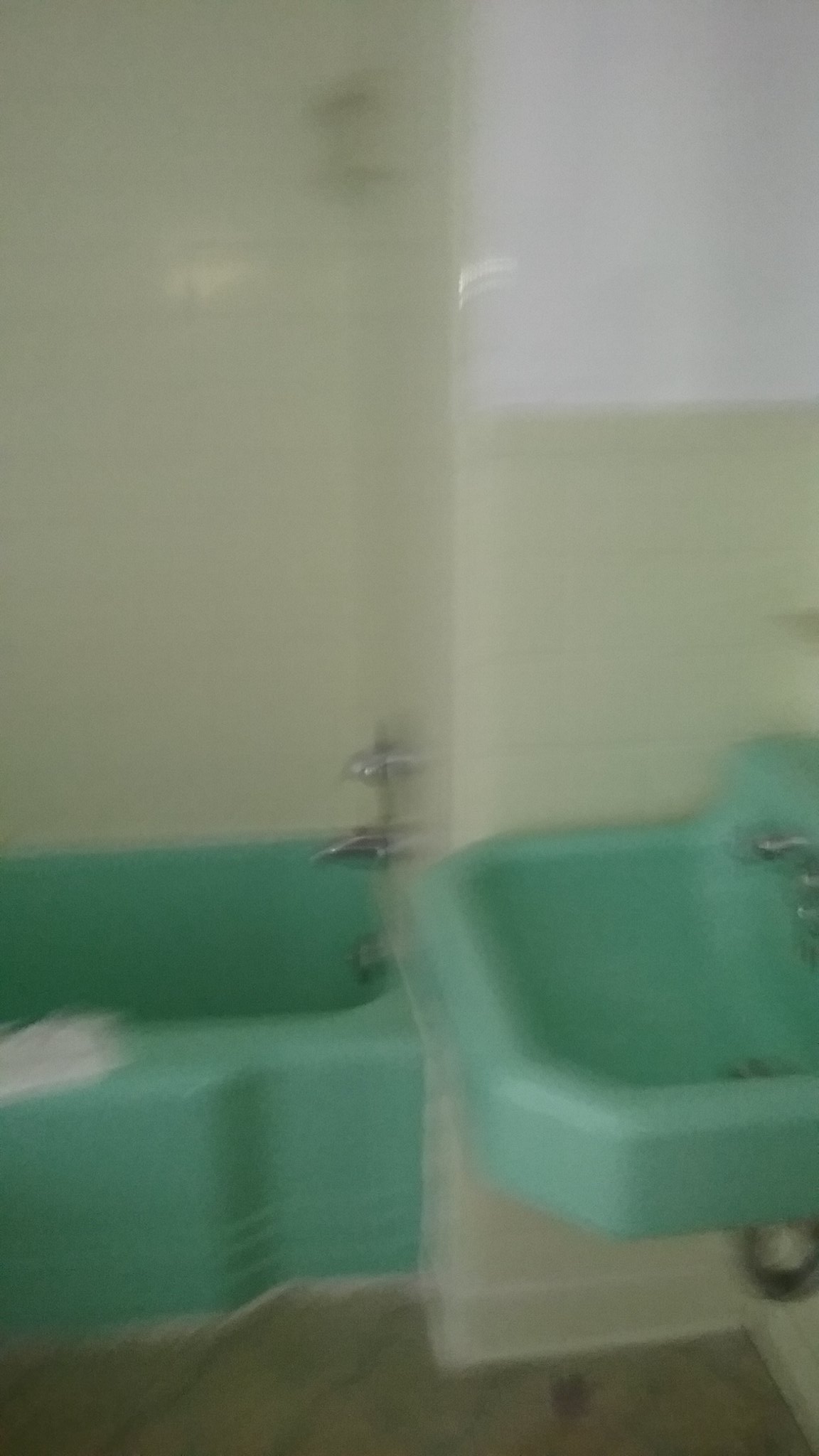This color photograph, though quite blurry, seems to depict a bathroom setting. The background features a greyish tiled wall with light reflecting off of it, particularly noticeable in the upper right section. The floor has a brownish grey tone. On the right side of the image, a green sink is visible, wall-mounted with a tap in the middle and possibly a plug cord and a pipe underneath. The tiles continue beneath the sink. To the left, a green bathtub is discernible, with taps situated on the wall at the center of the picture. A small white object rests on the rim of the bathtub, just to the left.